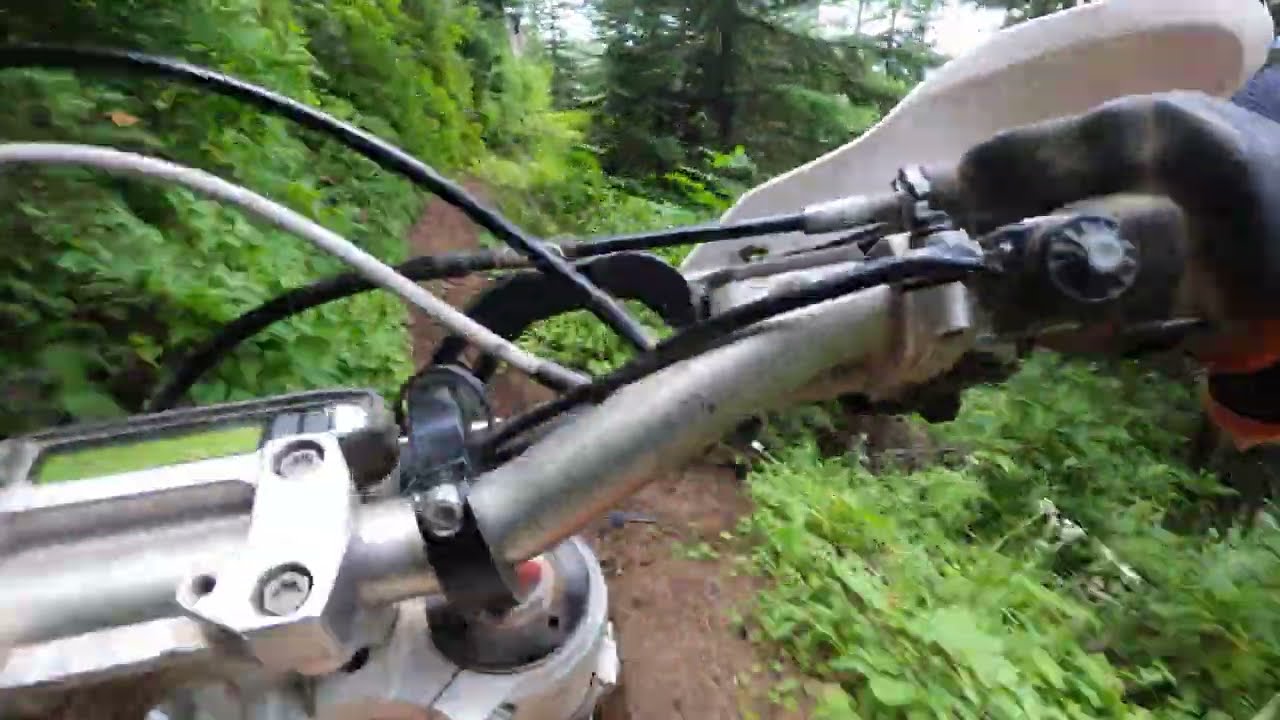The image is a rectangular photograph, almost twice as wide as it is tall, capturing the viewpoint of someone riding a motorcycle or motorbike along a narrow, muddy dirt path. The handlebars dominate the foreground, displaying a mix of shiny silver metal and intertwined black and gray cables arching upwards and off to the left side of the image. A green screen, possibly a readout device, framed in gray and dark gray, is visible on the left handlebar, which also features a manual dial. A gloved hand of the rider can be seen gripping the handlebars, adding to the sense of motion. The path itself, muddy and rugged, winds from the bottom center of the image, veering slightly to the left before disappearing into the dense vegetation. The background is filled with a rich array of greenery, including shrubs and evergreens, giving way to a bright sky that peeks through the canopy of trees. The day appears sunny, enhancing the vividness of the green foliage and casting a bright light over the entire scene.